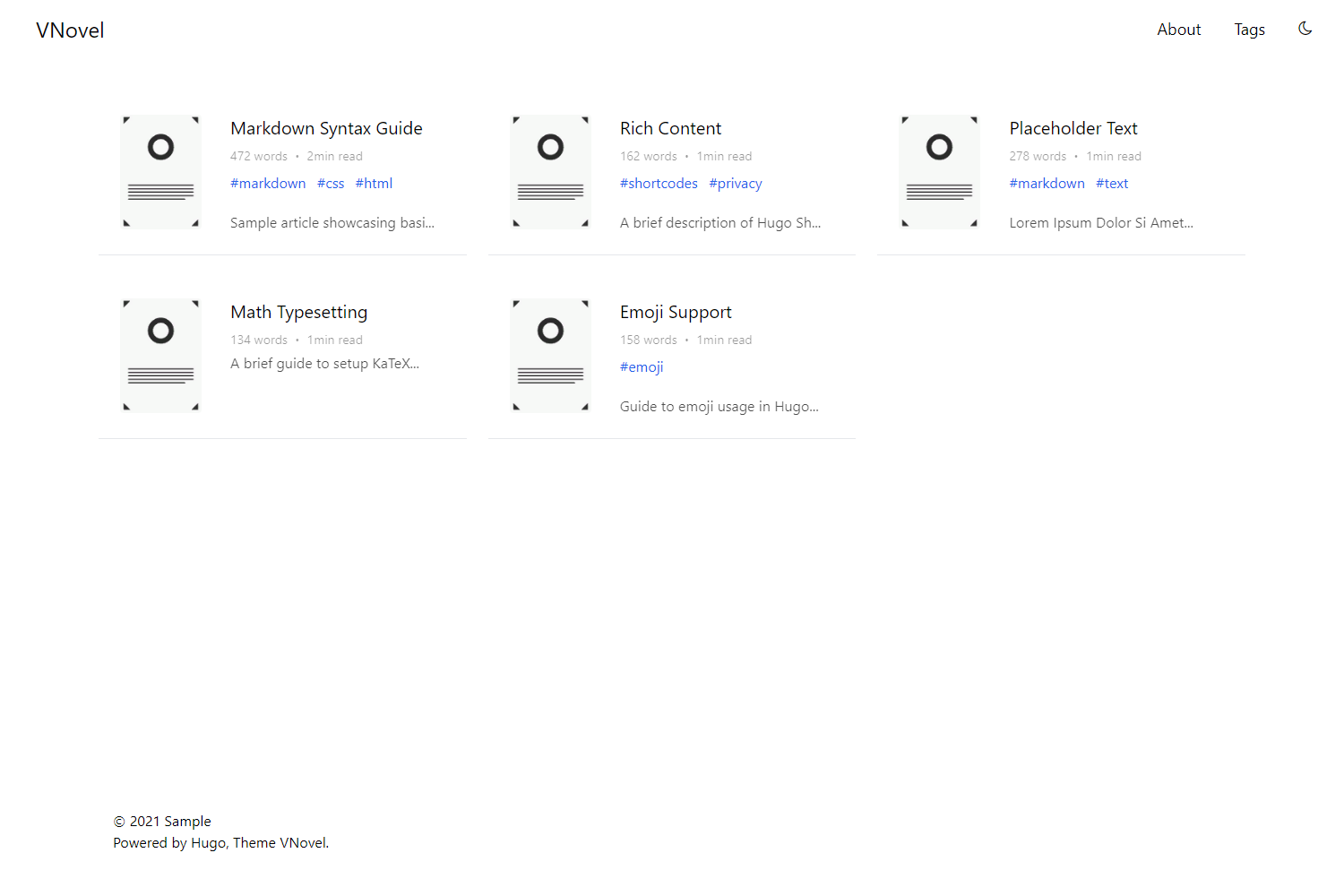The image depicts a web page titled "V-Novel," which appears to be a guide for using Markdown syntax. The page lists several short articles, each with brief descriptions, word counts, and estimated reading times. 

- **"Markdown Syntax Guide"**: 432 words, estimated reading time of 2 minutes. The article title is highlighted in blue and is described as showcasing basic Markdown, CSS, and HTML.
- **"Rich Content"**: 162 words, estimated reading time of 1 minute. Highlighted hashtags include #privacy. 
- **"Placeholder Text"**: 278 words, estimated reading time of 1 minute. Key hashtags are #Markdown and #text.
- **"Math Typesetting"**: 134 words, estimated reading time of 1 minute. The description mentions a brief guide to setting up KText.
- **"Emoji Support"**: 150 words, estimated reading time of 1 minute. The content guide is related to emoji usage in Hugo and is tagged #emoji.

Each article listing is accompanied by an icon resembling a page with a circle at the top and horizontal black bars representing text. 

Additional features on the page include navigation links in the top-right corner labeled "About," "Tags," and a "Late or Day" option. In the bottom-left corner, there's a footer indicating "© 2021, Powered by Hugo, Theme by V-Novel."

Overall, the webpage serves as a resource for entry-level writers to understand and apply Markdown syntax in their writing projects.